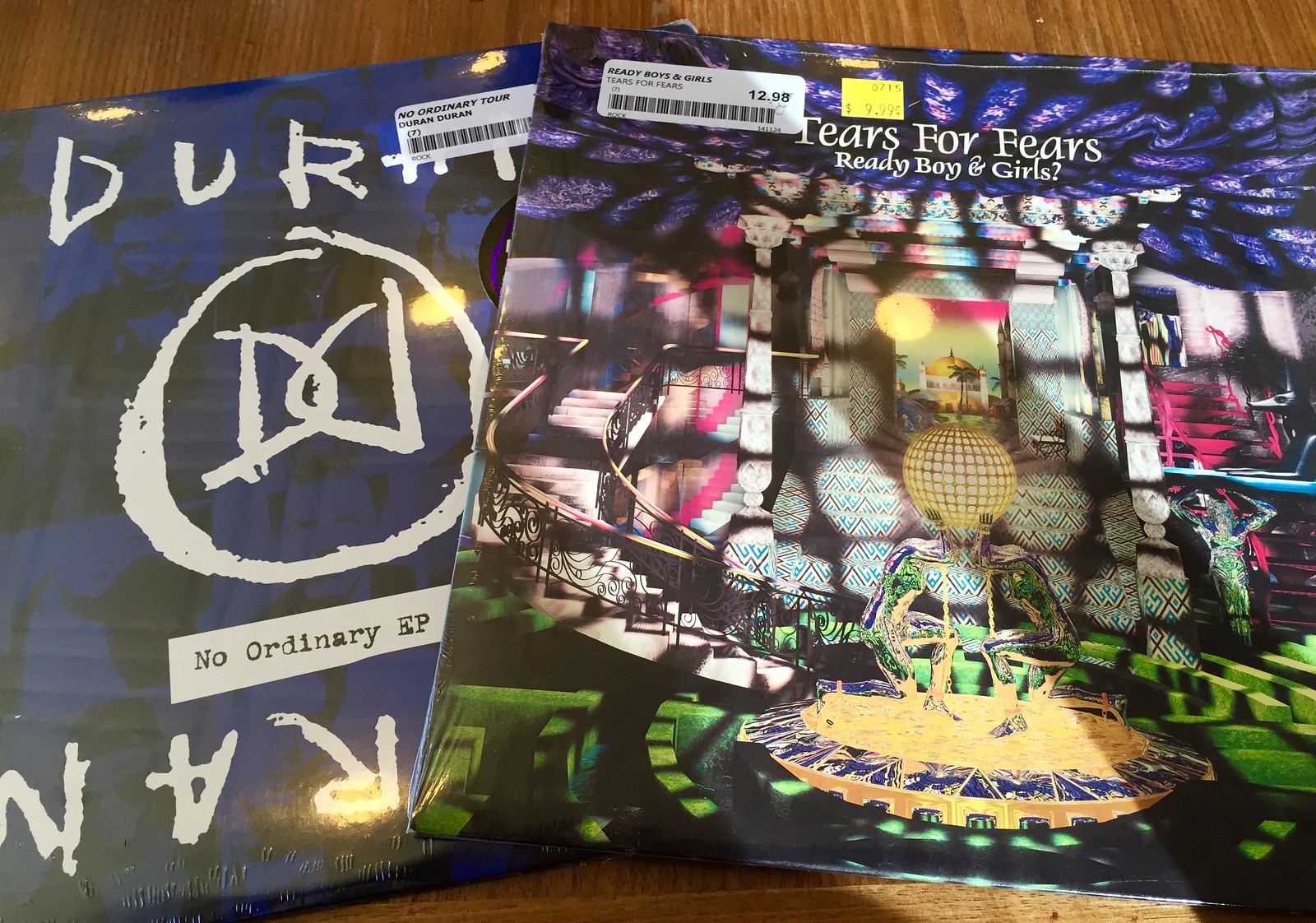The image showcases two vinyl album covers displayed on a wooden surface, bathed in light. The top-right cover is "Ready Boy and Girls" by Tears for Fears, while beneath it on the left lies "No Ordinary Tour" by Duran Duran. Both albums are still in their wrapping. The intricate album art of "Ready Boy and Girls" features what initially appears to be a table but is actually two figures in shiny, reflective latex holding up a lamp resembling a globe, set against a backdrop of a grand, alien-like mansion with spiral staircases and spotlights. The mansion’s ceiling glows purple, adding to the futuristic atmosphere. In contrast, the "No Ordinary Tour" cover is simpler, featuring a blue and black design with a handwritten "Duran Duran" and a distinctive logo in the center.